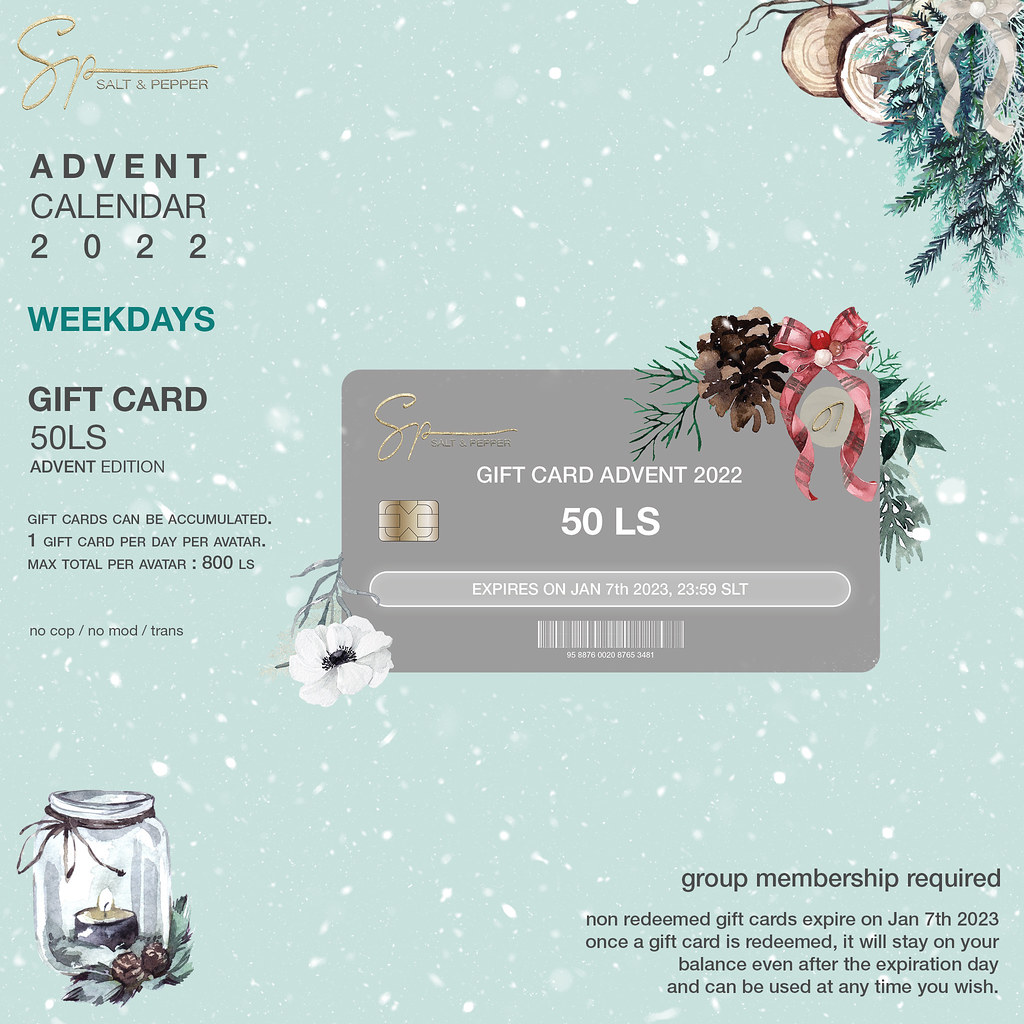This image is a digitally synthesized holiday-themed promotional advert featuring a teal blue background with white specks resembling snowflakes. In the center-right, there's a cartoonish, dark gray credit card. The card displays "Gift Card Advent 2022" in white text, "50 LS" beneath that, and "Expires on Jan 7th, 2023 23:59 SLT" below, alongside a white barcode. Holiday decorations adorn the card, including pine needles, pine cones, a red bow on the top right, and a white flower on the bottom left. The top right and bottom left corners of the image parallel the card's artwork, embellishing the scene with green pine needles, white ribbons, holly leaves, and a cartoon candle in a glass jar. In the top left corner, the letters "SP" in gold cursive are displayed, followed by "Salt and Pepper." Directly below, black text reads "Advent Calendar 2022," with the word "Weekdays" in green text below that, and "Gift Card 50 LS Advent Edition" in black beneath. Further text specifies "Gift cards can be accumulated one gift card per day per avatar, max total per avatar: 800 LS," and "No Copy / No Modify / Transfer." The bottom right corner states "Group membership required. Non-redeemed gift cards expire on January 7th, 2023. Once a gift card is redeemed, it will stay on your balance even after the expiration date and can be used at any time."